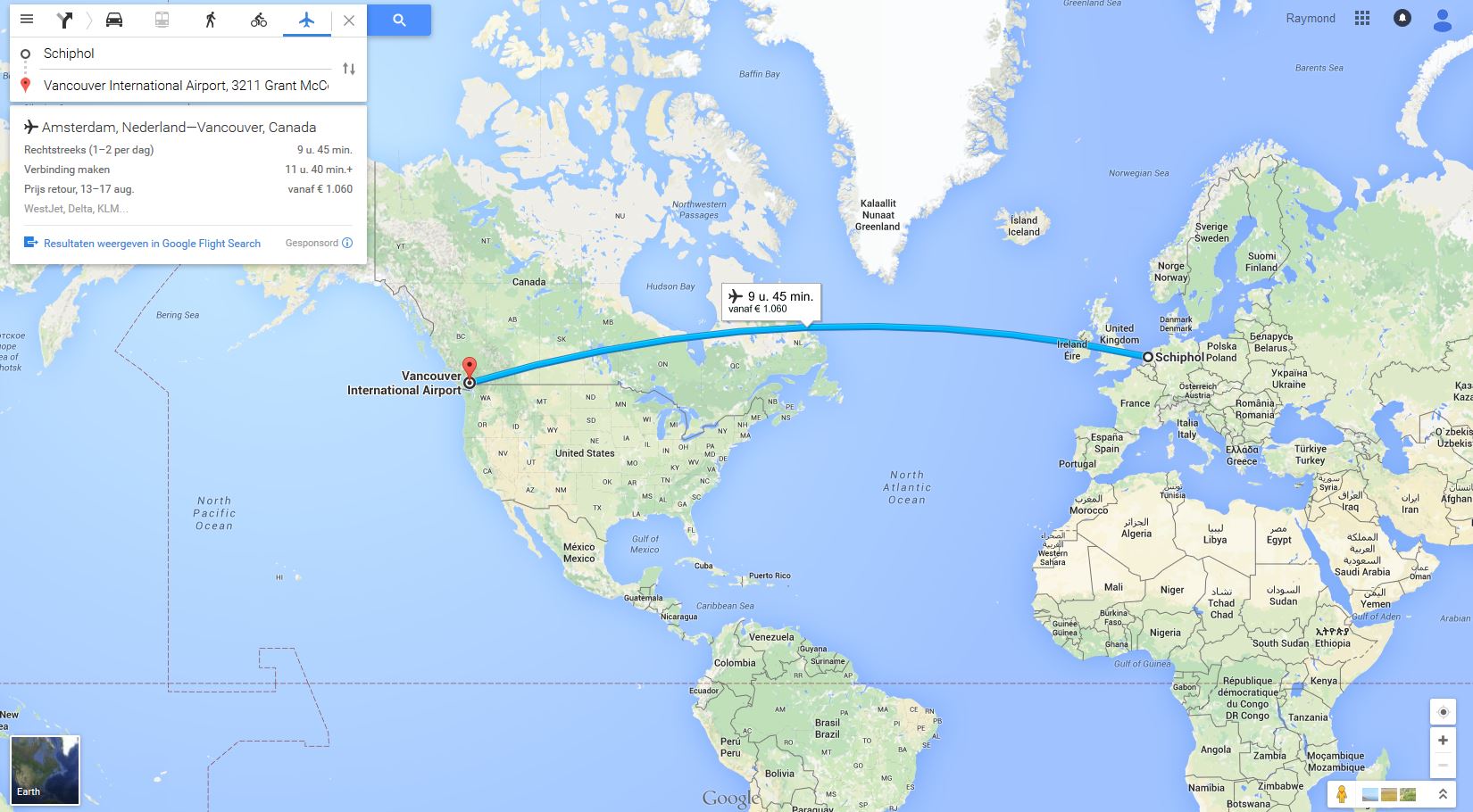A detailed screenshot from Google Maps, illustrating a flight route between Schiphol Airport in Amsterdam and Vancouver International Airport in Canada. The map prominently displays parts of North America and Europe, with countries clearly demarcated. Iceland and Greenland are visible near the top, surrounded by the expansive Atlantic Ocean. A distinct blue curved line traces the intended flight path across the ocean, highlighting the journey's trajectory. The estimated flight duration is marked as 1 hour and 45 minutes. Additionally, the iconic red arrow pointer from Google Maps indicates the final destination, providing a comprehensive visual guide for this transcontinental trip.